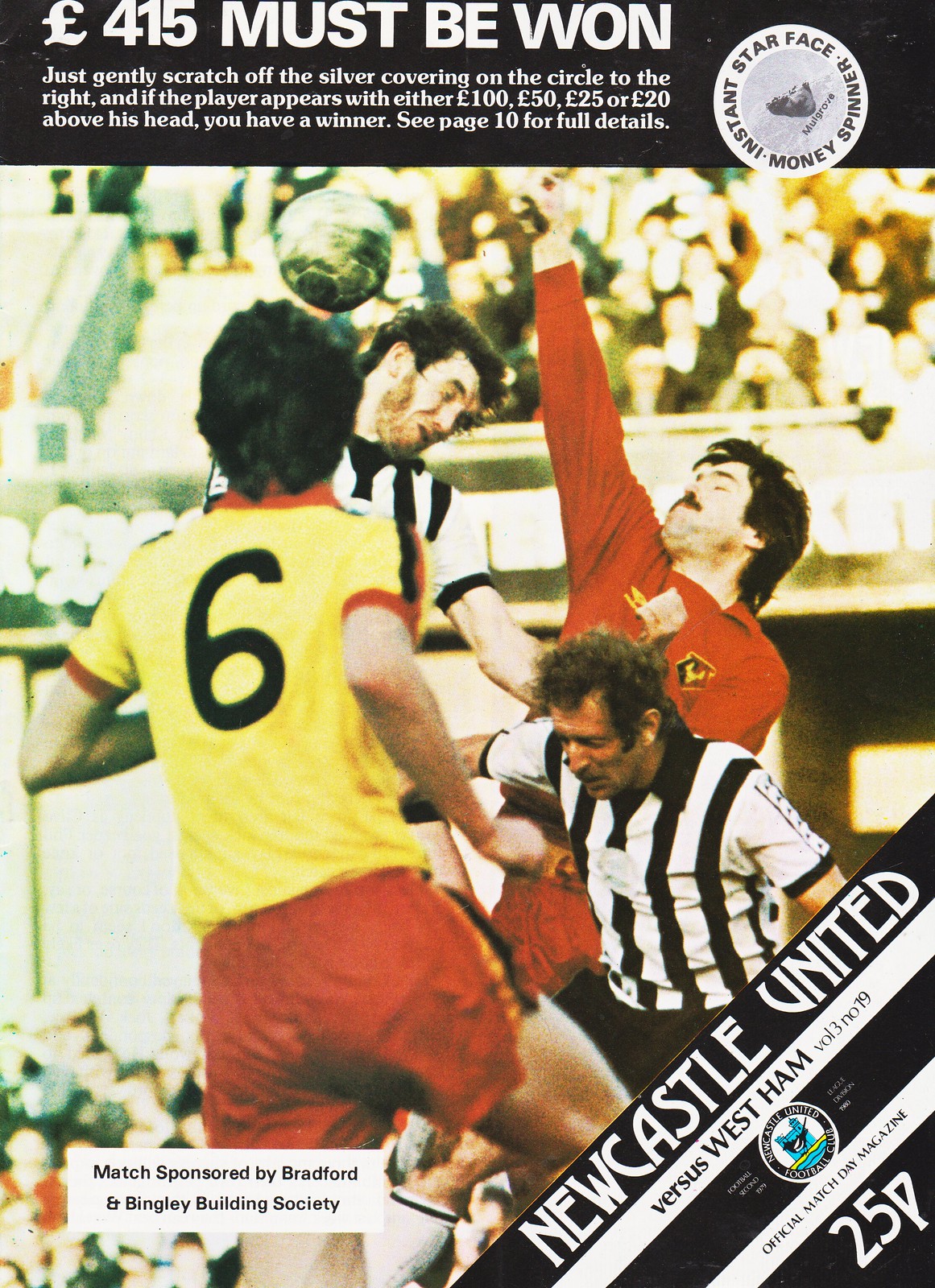This image is a scan of a football program, potentially featuring a promotional scratch-off ticket. At the top, white text on a black background declares, "415 pounds must be won." Below, instructions guide readers to "gently scratch off the silver covering on the circle to the right, and if the player appears with either 150, 25, or 20 pounds above his head, you have a winner," directing them to page 10 for full details. The main visual captures a dynamic soccer scene with three footballers—one in a yellow jersey and red shorts, another in a red jersey and red shorts—all attempting a header while two referees in white and black shirts intervene. The spherical object, presumably a soccer ball, is suspended in the air. The bottom left corner states "match sponsored by Bradford and Bingley Building Society," while the lower right announces "Newcastle United versus West Ham." Additional program details, including "25p," and "Volume 3 Number 19," designate it as an official match day magazine.